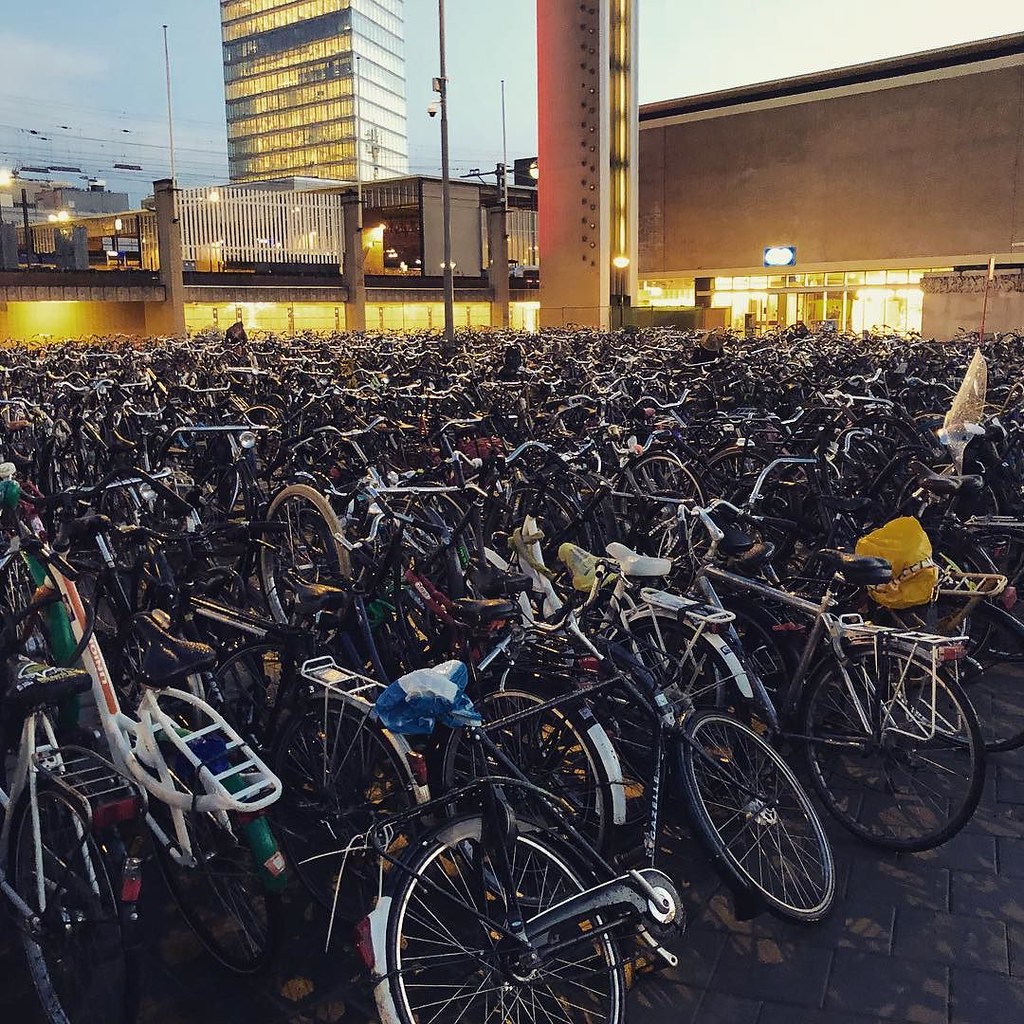This color photograph captures a crowded urban parking lot brimming with what appears to be hundreds of discarded bicycles. The eclectic array of bikes, characterized by metal frames, spokes, and handlebars in various colors, shapes, and sizes, spills across a blue tiled floor. Most of these bicycles resemble vintage road bikes, reminiscent of those commonly used for transportation in cities like Amsterdam. They are densely packed, with many aligned in the same direction but some perpendicular, creating a chaotic yet fascinating sea of cycles. In the immediate foreground, distinct features like a bike with a blue seat and another with a yellow rear holder stand out. The bicycles occupy a recessed area beneath a higher level, marked by a sidewalk and fence to the upper left. The background reveals a bustling urban environment with office buildings and a towering skyscraper. The office buildings’ windows glow with yellow lights, suggesting the setting sun of early evening, casting a light blue hue over the sky. From the upper right of the image, a storefront with large windows peeks out, adding another element to the urban scene. Overall, the image paints a vivid picture of this intriguing and somewhat chaotic bicycle graveyard, set against the backdrop of a city winding down as evening approaches.